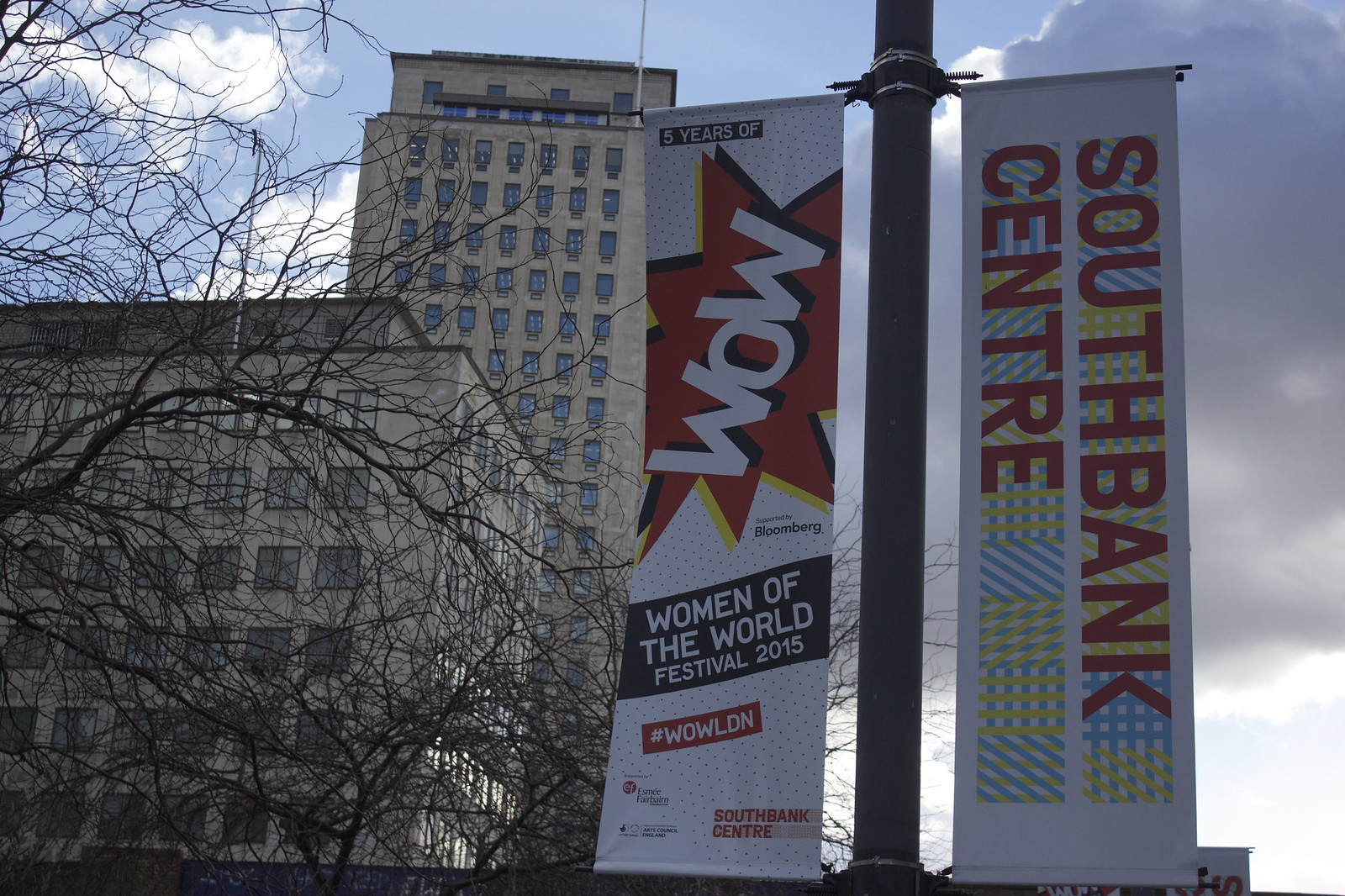An outdoor photograph captures two large gray buildings on the left, characterized by numerous windows and a uniform, concrete appearance. In front of these buildings, several leafless trees stand starkly against a cloudy sky, possibly indicating the season is fall or winter. The sky itself is dominated by heavy, dark clouds, although patches of blue are visible amidst the ominous cover.

To the right of the buildings, a black lamppost or metal pole supports two vertical signs. The sign on the left is predominantly white with red accents and reads "Five years of WOW!" – an advertisement for the Women of the World Festival 2015. The white letters are set against a red, starburst-like background, and the hashtag #WOWLDN is displayed in a red rectangle at the bottom.

The sign on the right, also white but with red, yellow, blue, and green accents, states "South Bank Centre" with the text oriented vertically in red letters. These signs are set against a backdrop of tree branches and urban architecture, further emphasizing the bustling atmosphere surrounding the South Bank Centre during this eventful time.